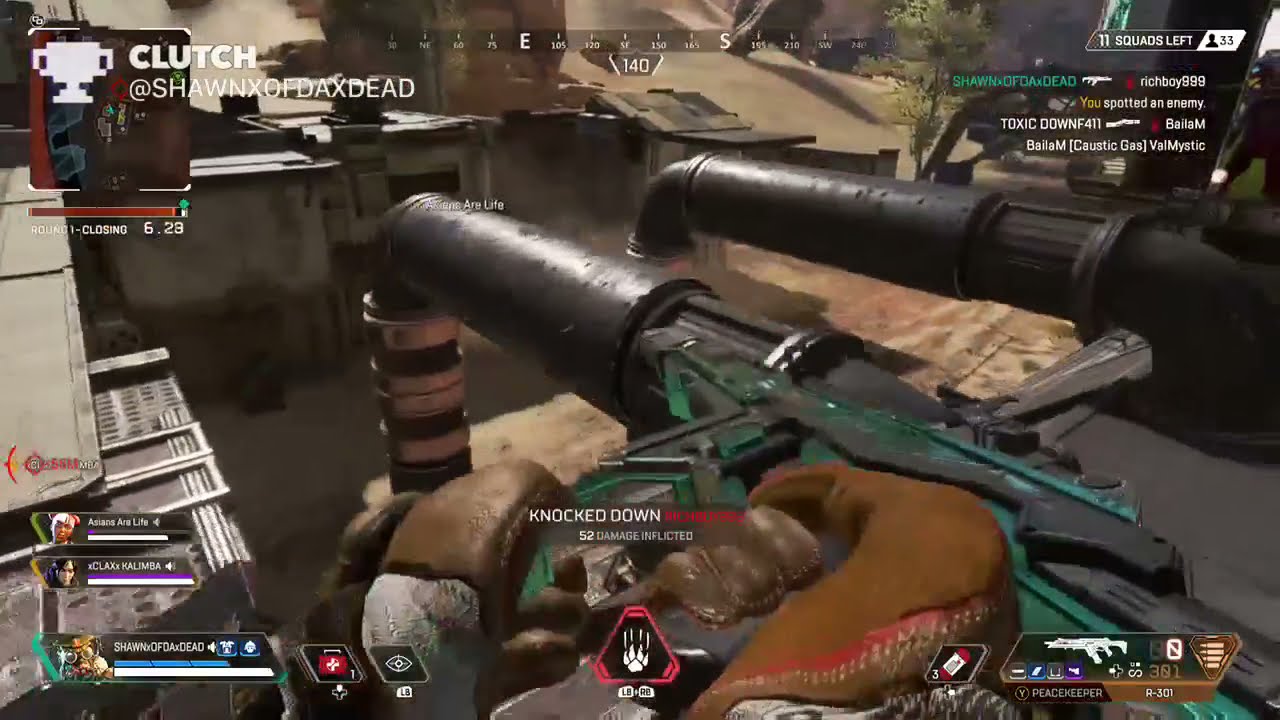The image is a highly detailed screenshot from a first-person shooter video game, reminiscent of titles like Call of Duty. The player character's hands, clad in brown gloves, are prominently extended from the bottom edge of the frame, gripping a green and black machine gun with a notably long barrel. The gun is held at a 90-degree angle to the right, with the left hand positioned near the magazine, suggesting that the player is in the process of reloading.

The heads-up display (HUD) is packed with information. In the top left corner, there is a mini-map that displays the player’s location, and adjacent to it, text details the current status of the game, noting events like kills and the remaining number of squads and players ("11 squads left. 33 people"). The text also includes names like "Clutch" and "Sean X of Dax Dead." A compass at the top center shows the player is moving east, while directly below the compass, statistics such as bullets remaining, “knocked down,” and “52 damage inflicted” are displayed.

In the lower left corner, there’s a life gauge and a button icon indicating a healing capability. Player names are mentioned here as well, though they are difficult to read. The lower right corner shows the ammunition count and grenade supply. The background features a sandy courtyard bordered by short buildings, lending a sense of a cluttered and chaotic environment on a platform overlooking this area.